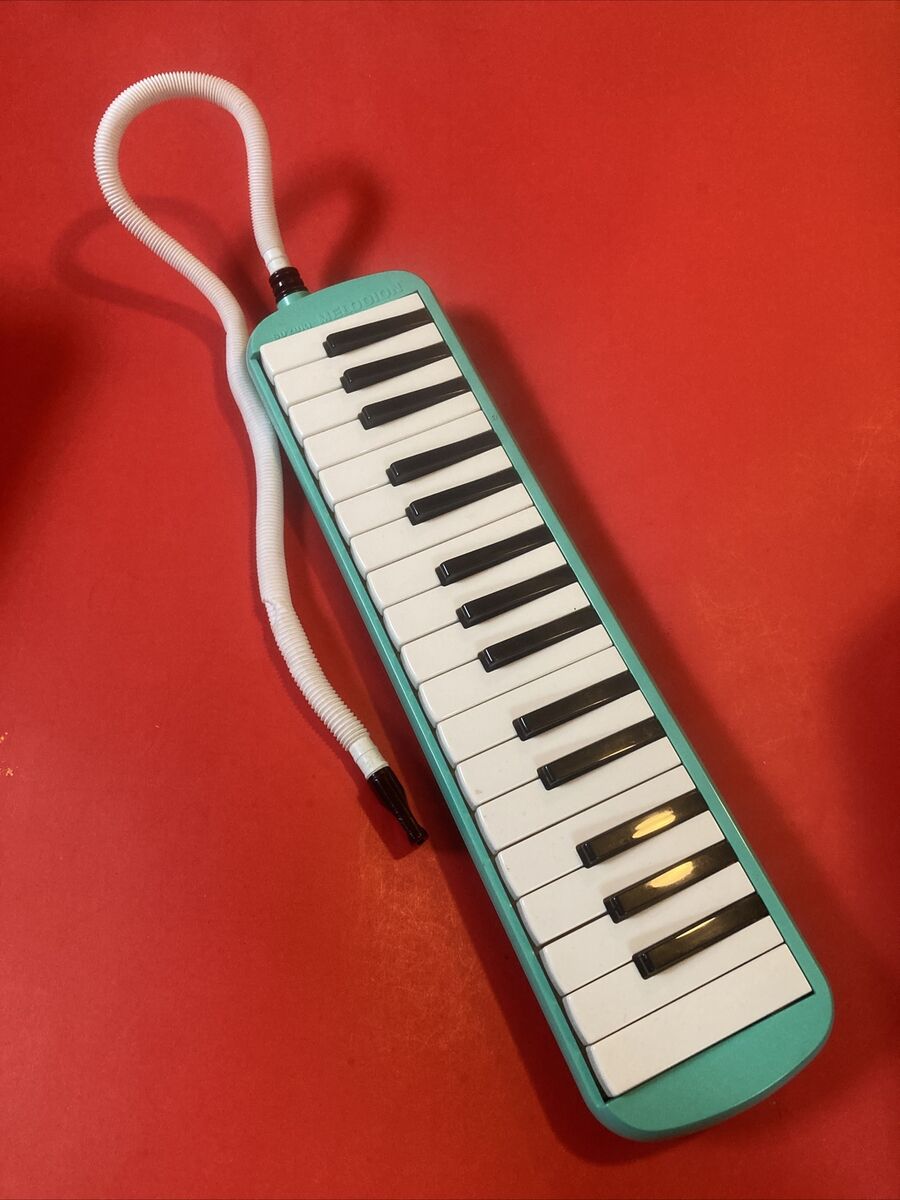The photograph depicts a close-up of a melodica, a portable keyboard instrument, set against a solid red background. The body of the instrument is a light teal or turquoise blue, with the familiar arrangement of black and white keys—specifically 19 white keys and 13 black keys. Prominently, the word "Melodian" is inscribed above the keys near the left where a white, flexible tube emerges. This tube, designed for blowing air into the instrument, curves gracefully downward and ends in a black pointed tip. The light source, though not visible in the image, casts distinct shadows to the right of the melodica and its tube. The shadows suggest additional, unseen objects partly visible as dark shapes in the top left and bottom right corners of the image.